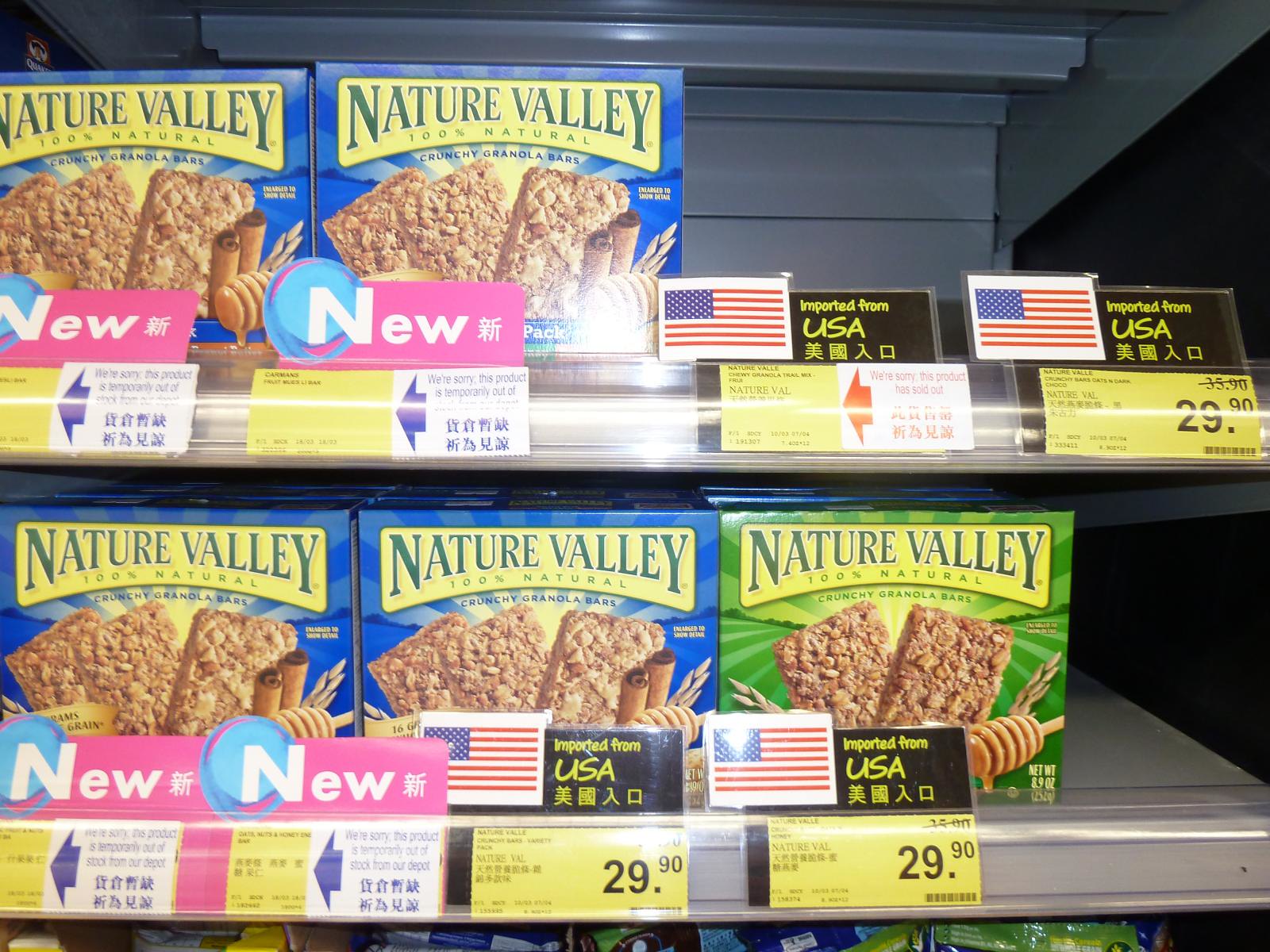In this image, we see two shelves in a supermarket displaying a collection of Nature Valley Crunchy Granola Bars. The focus is on the granola bars, which are mainly in blue boxes with a distinctive yellow section featuring the product name and images of the granola bars. There are also fewer green boxes present. The blue boxes display three granola bars on the packaging alongside a rolled-up cinnamon stick, suggesting a cinnamon flavor, whereas the green boxes show two granola bars with a honey wand, indicating a honey flavor. Several price tags are visible; they are rectangular, half yellow and half white with blue text in both English and Asian characters, possibly Chinese or Japanese. The price tags indicate $29.90, although the currency is unspecified. Some empty slots on the shelf have signs saying, "We're sorry, this product is temporarily out of stock," along with an image of an American flag and the phrase "imported from USA," suggesting that the supermarket is located outside of the United States.